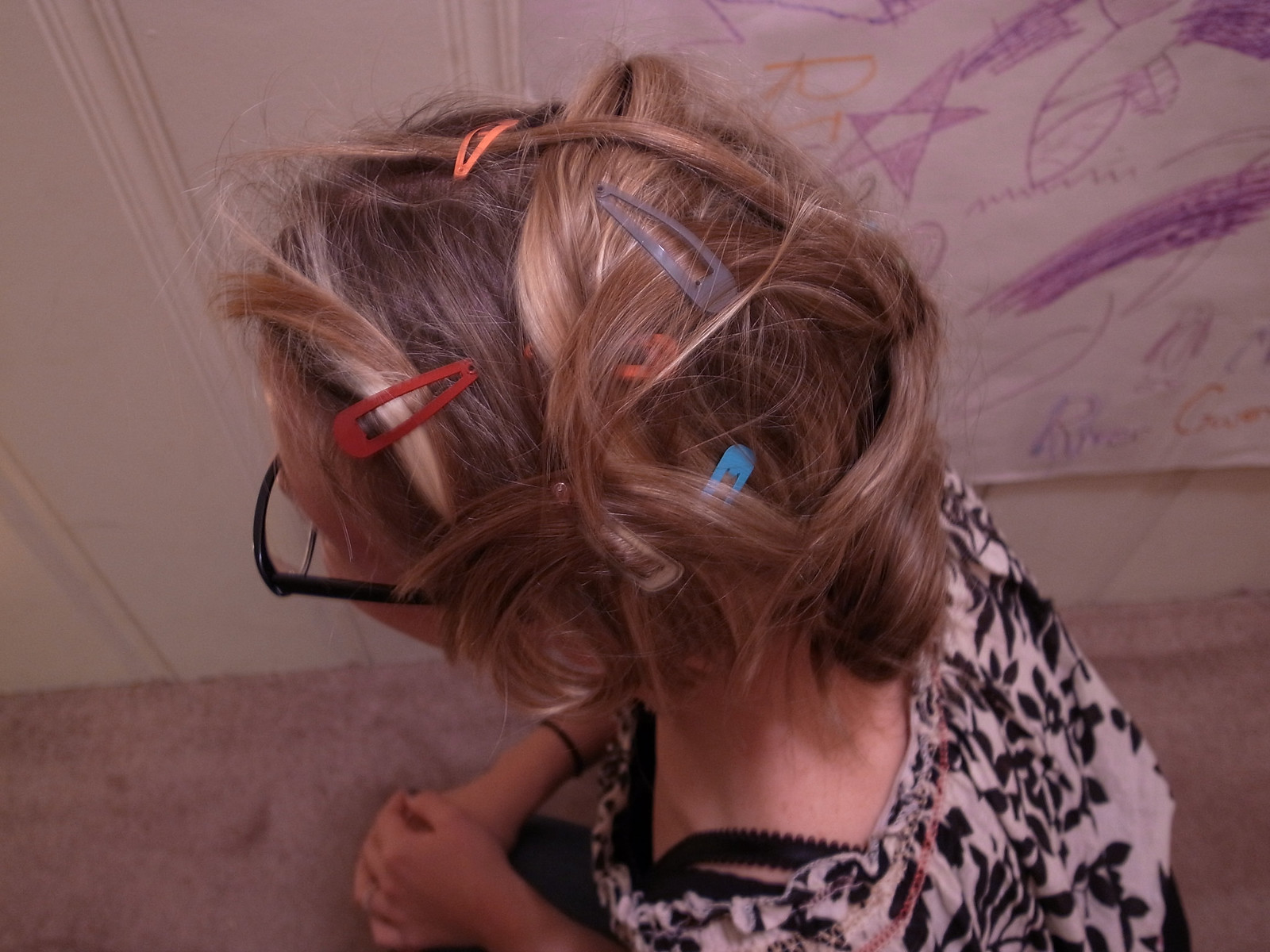This image captures an aerial view of a woman sitting on a pinkish carpet, viewed from above or slightly from the left side, giving a clear profile from her shoulders to her waist. She has short, brunette hair with dishwater blonde highlights, adorned with numerous hair clips in various colors: red, bright neon orange, light blue, gray, and an additional orange one partially hidden under her hair. These clips seem randomly placed, perhaps by a child. She wears black glasses with clear lenses, a black and white shirt featuring a black motif of leaves, and a visible black bra strap on her left shoulder. Her right wrist sports a black bracelet. The background shows a beige paneled wall with a large piece of paper covered in childlike drawings and scribblings, mainly in purple and orange, including stars, squiggles, little faces, and the word "go." Her hands rest on her knee, emphasizing a casual and intimate scene.